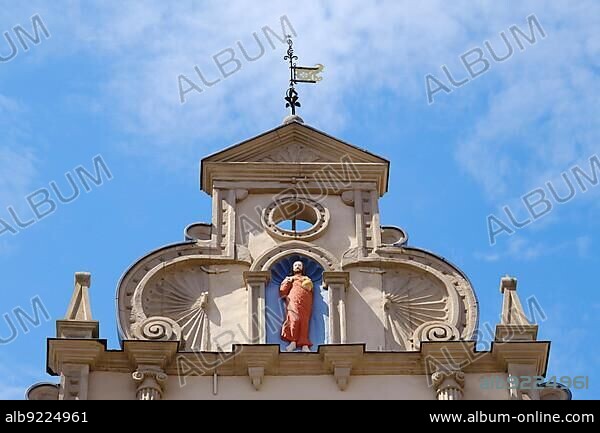The image depicts an ornate white stone shrine captured from an upward angle, showcasing detailed architectural elements. The central focus is a rounded wall rising to a triangular peak. At the apex, a metal bar extends upward, resembling a flagpole or weathervane. Below, nestled in a carved-out blue background, is a statue of a barefoot man with pale skin, brown hair, and a brown beard, donning a red robe. This statue appears to represent a religious figure and is depicted in motion as if walking. The backdrop features a clear blue sky adorned with very light clouds. A black strip at the bottom of the image bears the watermark, "ALBUM," with the code "ALB 922-4961" on the left and the web address "www.albumonline.com" on the right.